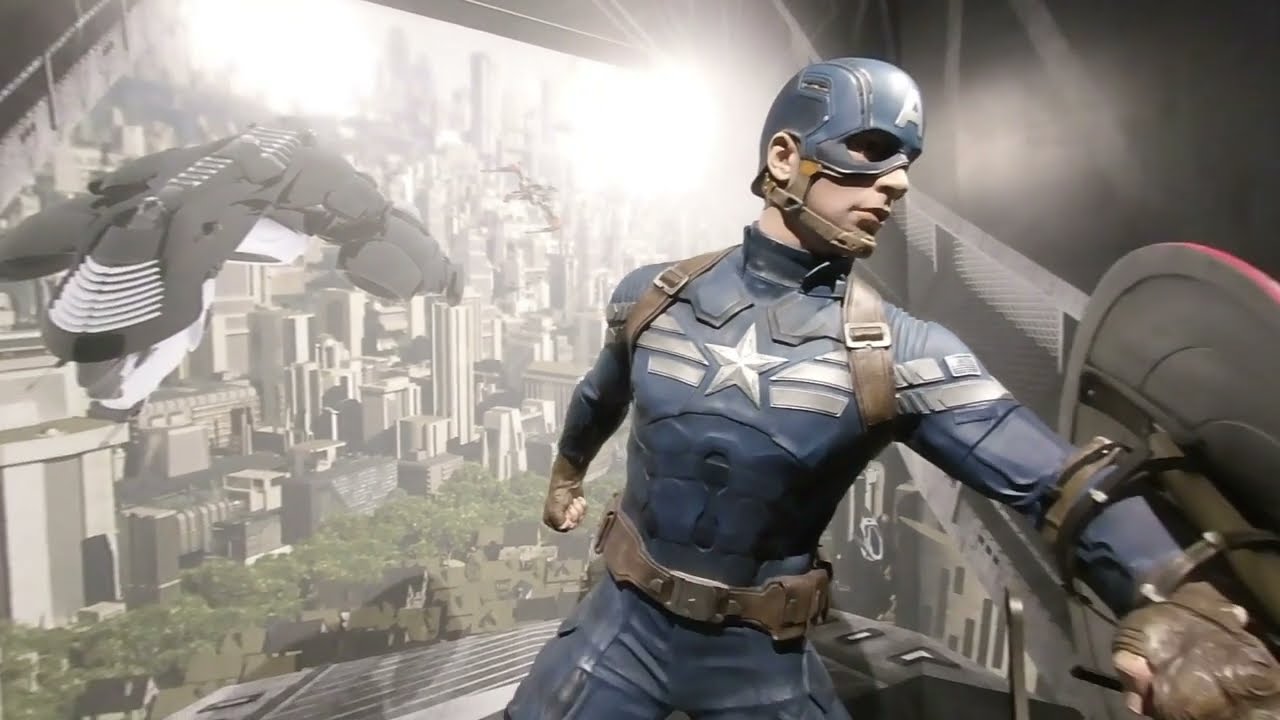In this highly detailed, computer-generated image, we see a lifelike depiction of Captain America in an action pose, seemingly set within an aircraft. Captain America, in his standard blue uniform adorned with a star on his chest and stripes nearby, stands closest to the center of the image. He has a shield strapped to his left arm, and his right arm is pulled back as if preparing to punch. His costume also includes brown leather gloves, a belt, and straps over his shoulders, along with a blue leather helmet secured by a brown strap.

To the right side of the image, Captain America appears particularly muscular, with attention to lifelike details in his Caucasian skin and the reflective light on his outfit and shield. In the background, an open bay door reveals a cityscape beneath and an incoming black craft with forward-pointing wings, suggesting an impending confrontation. The setting, illuminated by lights above, gives the impression of an indoor scene, possibly a museum or a hangar, enhancing the dramatic and heroic atmosphere of the visual.